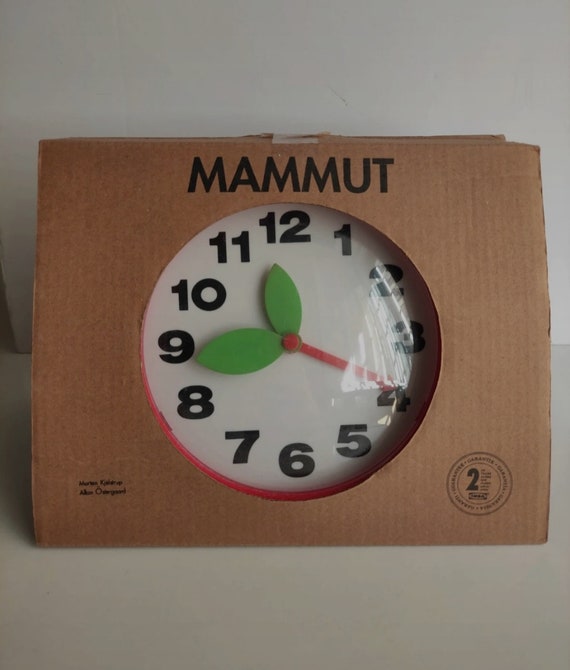The image displays a clock still encased in its original packaging, which is made of brown, textured cardboard. At the top of the cardboard, in bold black text, is the brand name "MAMUT." The packaging features a round die-cut hole through which the clock face is prominently visible. The clock face is white with plain black numbers from 1 to 12 and has a distinctive design element: instead of multiple hands, it has a single red stem, akin to a plant stem, with two green metallic leaves attached, seemingly functioning as additional clock hands. The bottom left of the packaging contains some small, unreadable text, while the bottom right includes a seal that has the number "two" and some smaller text, also too small to discern. The clock itself has a red border that frames the clock face, complementing its unique design. The packaging appears to be unopened and is placed against a beige backdrop.